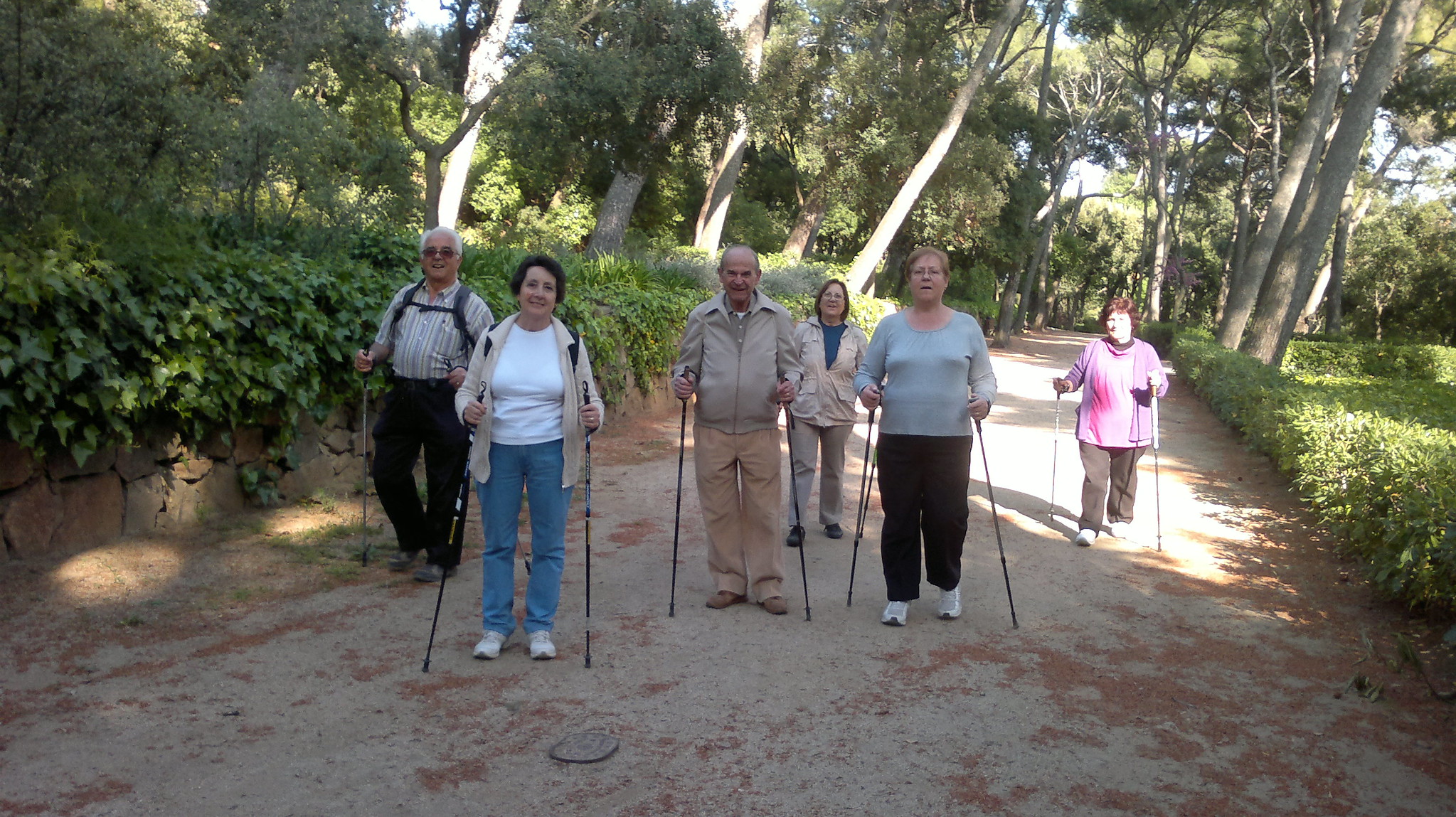In this vivid, color photo taken horizontally, a group of six people stands on a well-maintained, wide dirt trail in a park-like setting or the wilderness. The trail is dotted with dried brown pine needles and lined with leafy vegetation and tall trees. Everyone appears to be in their 60s or 70s and is carrying a pair of black hiking sticks, indicating they are likely on a casual, outdoor hike. 

Starting from the left, an older man with white hair wearing sunglasses, a striped shirt, and black pants pulled high on his waist is seen sporting a backpack. To his right, a woman in a white shirt, blue jeans, and a light yellow cardigan smiles brightly. 

Central in the group, a balding man with fair skin is dressed in a light gray jacket and khaki pants. Just to his right, a woman stands slightly behind him, donning a tan coat with beige pants and a blue undershirt; she has brown hair. 

Next to her, another woman wears a light blue top and black pants, with glasses perched on her face and light brown hair framing it. On the far right, a woman, partially obscured and slightly distanced, has donned a pinkish-red top and gray pants and has reddish-brown hair.

The trail is bathed in daylight, and the group’s casual outdoor attire completes the atmosphere of a pleasant day spent hiking together in nature.